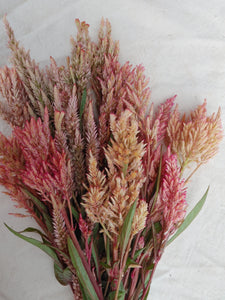In this detailed image, a flat bouquet of flowers is showcased against what seems to be a light gray or white backdrop, notable for its streaky texture. The arrangement prominently features a diverse mix of colors, including vivid shades of pink, yellow, pale peach, and light brown, complemented by substantial green foliage. The flowers appear to be clumped together, creating an effect where the petals resemble colorful stems or stalks, some exhibiting pink tips. While it's unclear if the bouquet is real or artificial, the flowers and leaves lay in a seemingly arranged manner, possibly on a table or a white tablecloth, as no vase is visible in the image. The overall scene is devoid of text, people, or additional objects, focusing solely on the vivid display of the flora against the muted background.